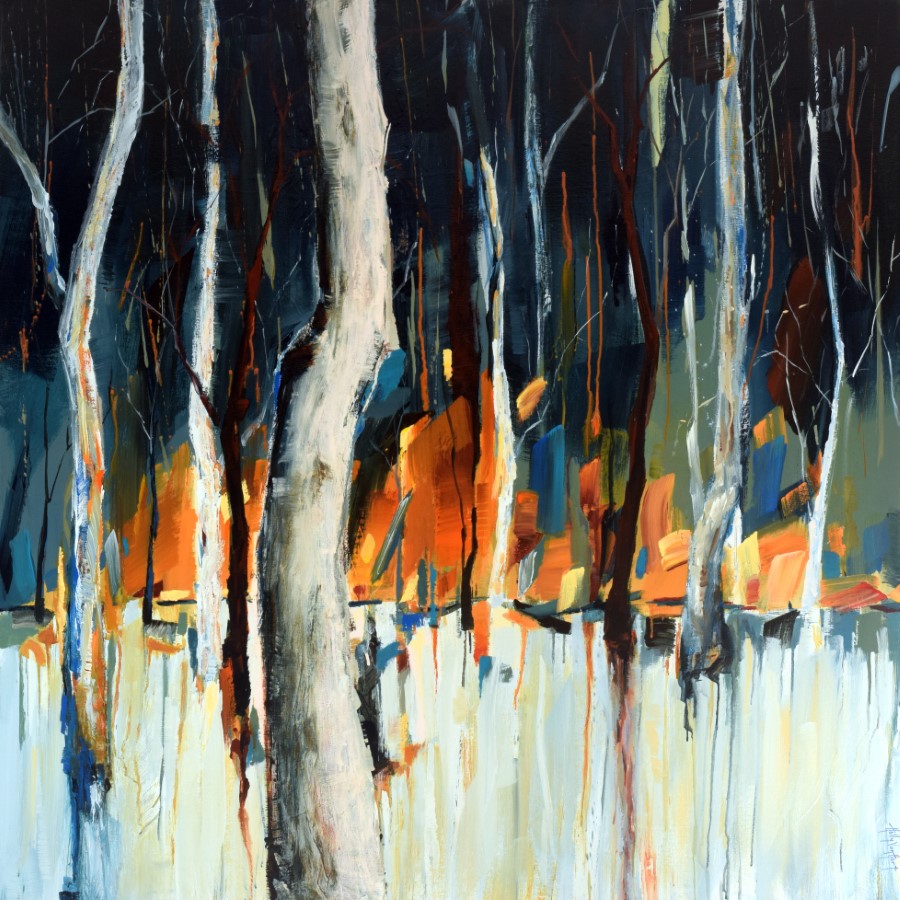The painting captures an abstract, outdoor landscape featuring a variety of white and grayish tree trunks, reminiscent of birches, with leafless branches weaving through the scene. Scattered throughout the image, these trees create a dense, wooded area. Notably, the trees in the foreground are more detailed, while those in the background blur into abstraction. Adding depth and contrast, vibrant hues of orange, teal, and medium blues splash across the canvas, particularly near the middle, where a fiery burst of orange stands out, suggesting something bright and vibrant occurring in the background. The lower section of the image features a white compound wall-like structure that fences in the trees and separates them from orange shrubs below. The sky, painted pitch black, indicates nighttime, contributing to the dramatic and mysterious ambiance of the piece. Overall, the painting merges realistic tree depictions with abstract color applications, creating a rich and interpretable landscape.